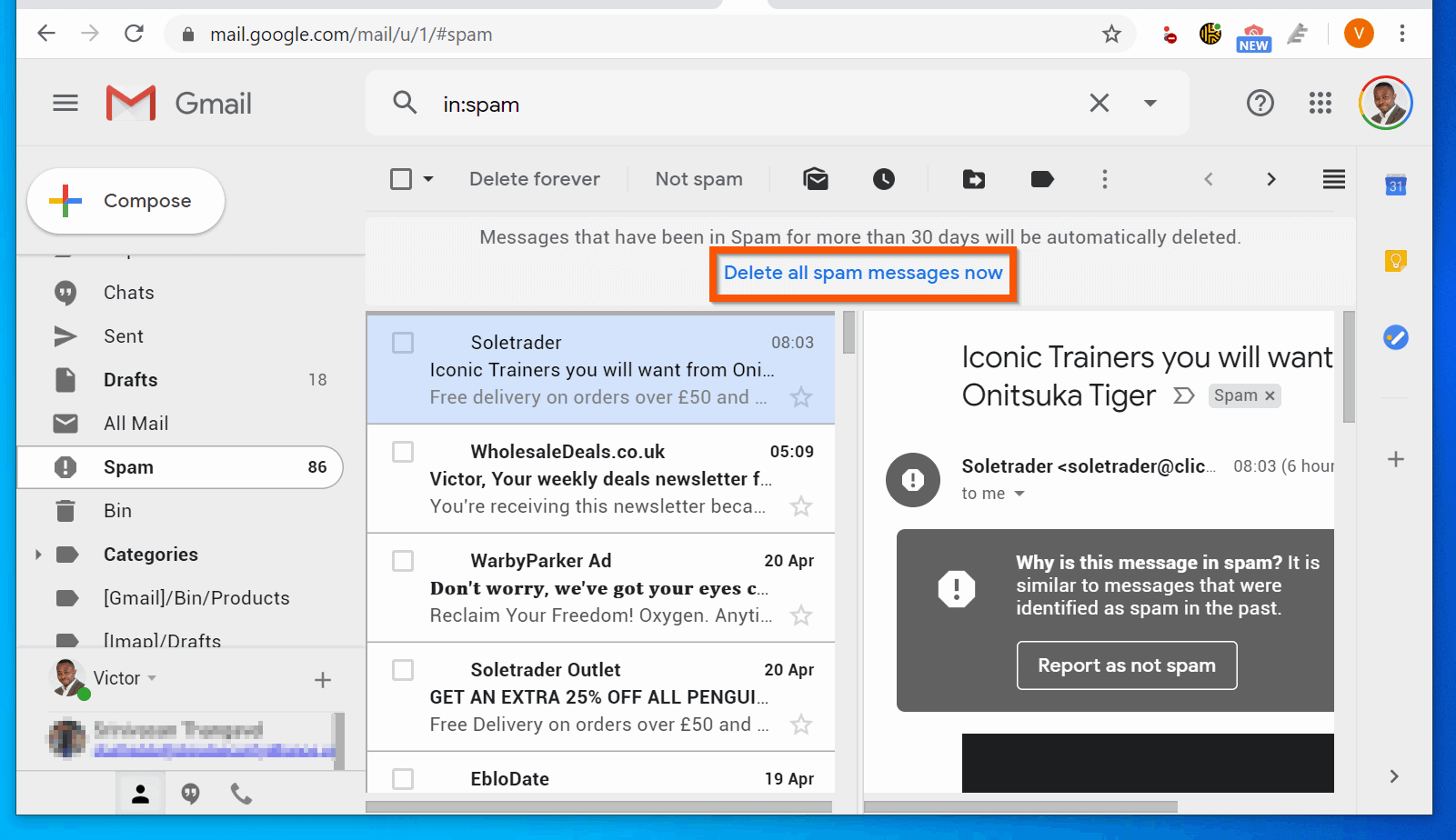Screen capture of the Gmail homepage, displaying an opened account. The left column showcases various categories, starting with a prominent red "M" icon followed by the word "Gmail" in gray font. Below this, a white oval button labeled "Compose" is visible. The folder list beneath includes icons and labels for "Chat," "Sent," "Drafts," "All Mail," "Spam," "Bin," "Categories," and a partially visible item labeled "gmail/bin/products," with the last entry obscured by an overlay. 

The selected category is "Spam," containing 86 items. On the right, the layout includes a column listing emails and a preview pane to the right. The foremost email is from "Sole Trader" with the subject "Iconic trainers you'll want for." The top portion of the screen features a red rectangular outline with the message "Delete all spam messages now," which is highlighted, indicating an instructional intent on how to clear out the spam folder.